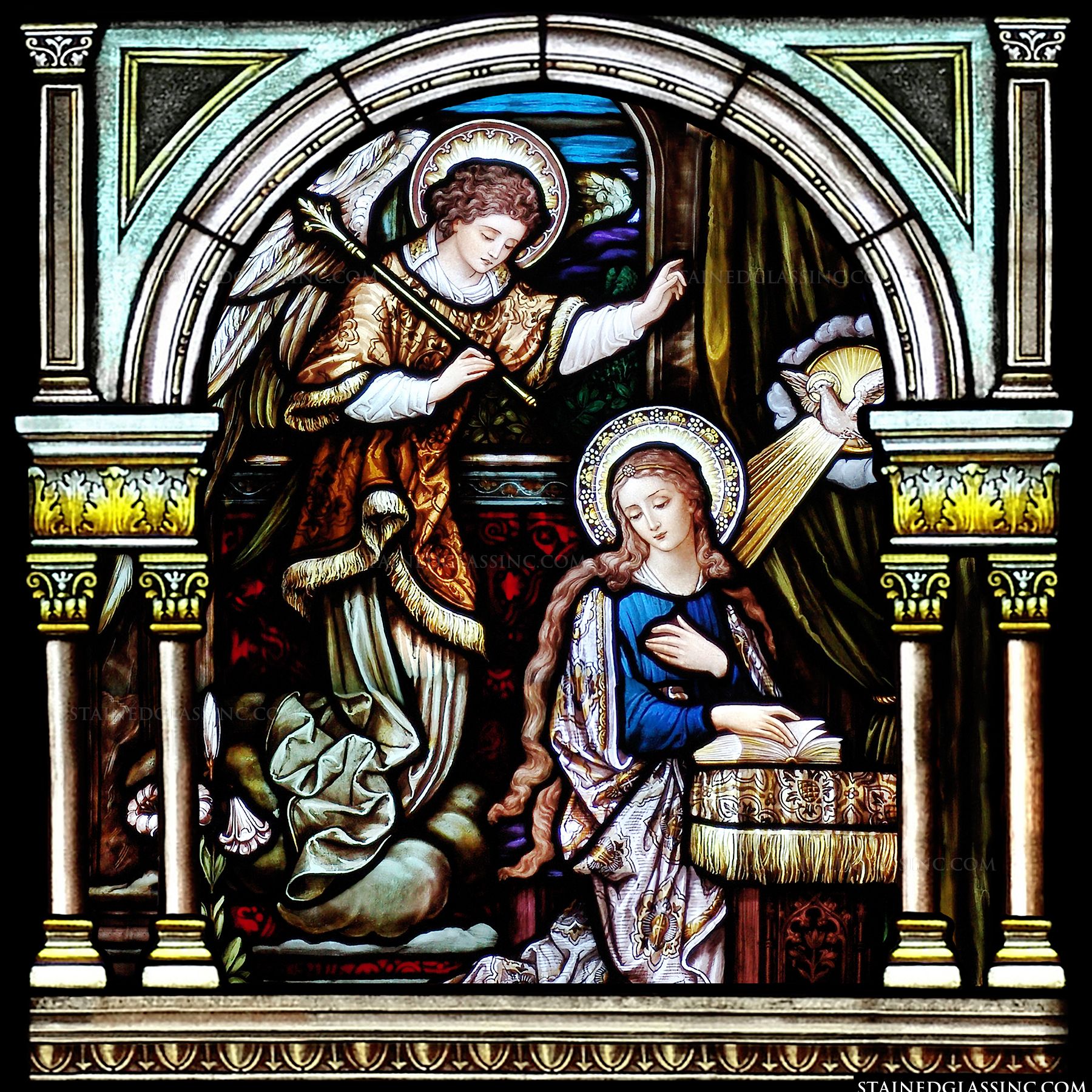The image depicts a religious scene rendered in a two-dimensional, possibly stained glass or painted style, characterized by dark, black outlines and an ornate, cathedral-like aesthetic. At the center is Mother Mary, adorned with a decorated white halo encircling her head. She has long, curly, brown hair and is garbed in a blue dress with a white and red shawl over her shoulders. Mary is kneeling on a striped ottoman with beige fringe, intently reading an open book placed atop it, her left hand helping to hold it open while her right hand rests on her chest.

Above Mary is an angel with white, feathered wings and a similarly embellished white halo. The angel has curly hair and is dressed in a brown and white robe. In one hand, the angel holds a staff or rod, while the other hand is outstretched. The scene is set under a prominent white arch supported by two columns on each side, enhancing the sacred and historical feel of the artwork. Adding to the divine atmosphere, there is a dove emitting light, positioned to shine upon Mary from the right side.